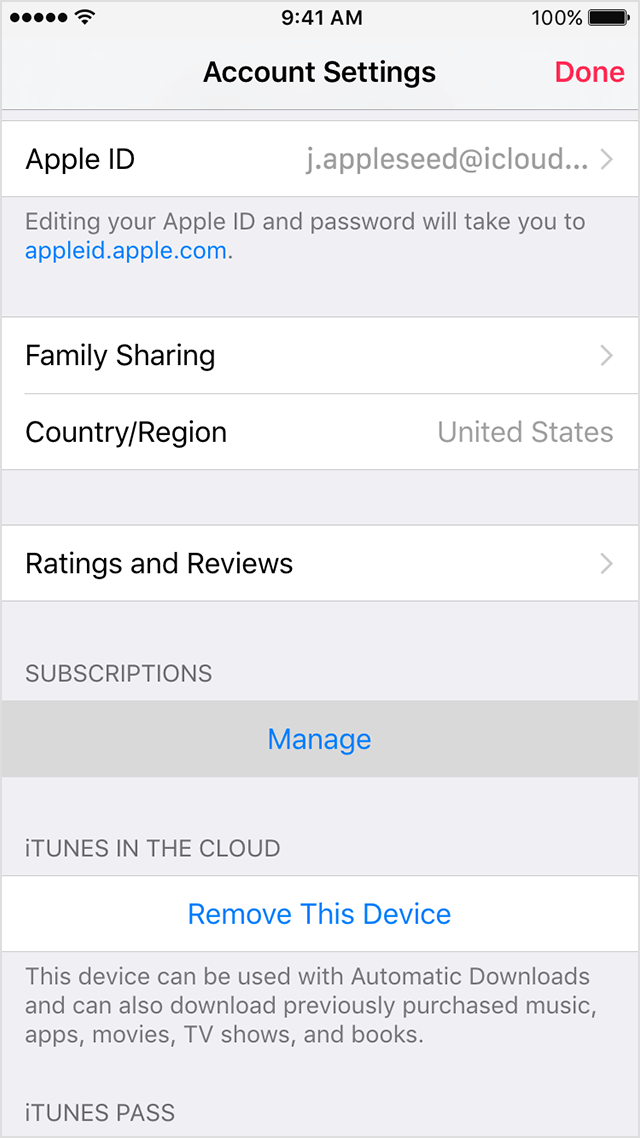The image portrays a smartphone screen, which is fully charged at 100% and shows the time as 9:41 AM. In the top left corner, there are four large dot indicators, signifying sound settings. The screen primarily displays Apple ID details, set against a white background with the name initial "J." 

Below this, it prompts the user to edit Apple ID and password by visiting "appleid.apple.com", highlighted in blue, signifying it is a clickable link. The next section is labeled "Family Sharing," followed by "Country/Region: United States." These sections are separated by gray divider bars.

Further down, another section titled "Ratings and Reviews" appears, with the word "Subscriptions" in gray underneath it. The subsequent darker gray section contains the option "Manage" in blue text, indicating an actionable link.

The following area is marked "iTunes in the Cloud" and is divided by another gray bar. Then, in a white section, it states "Remove this device" in blue lettering, suggesting another clickable option. The final gray section explains that this device can be used for automatic downloads and the retrieval of previously purchased media, including music, apps, movies, TV shows, and books.

At the very bottom left of the image, it mentions "iTunes Pass" and at the top, in conspicuous red text, is the word "Done."